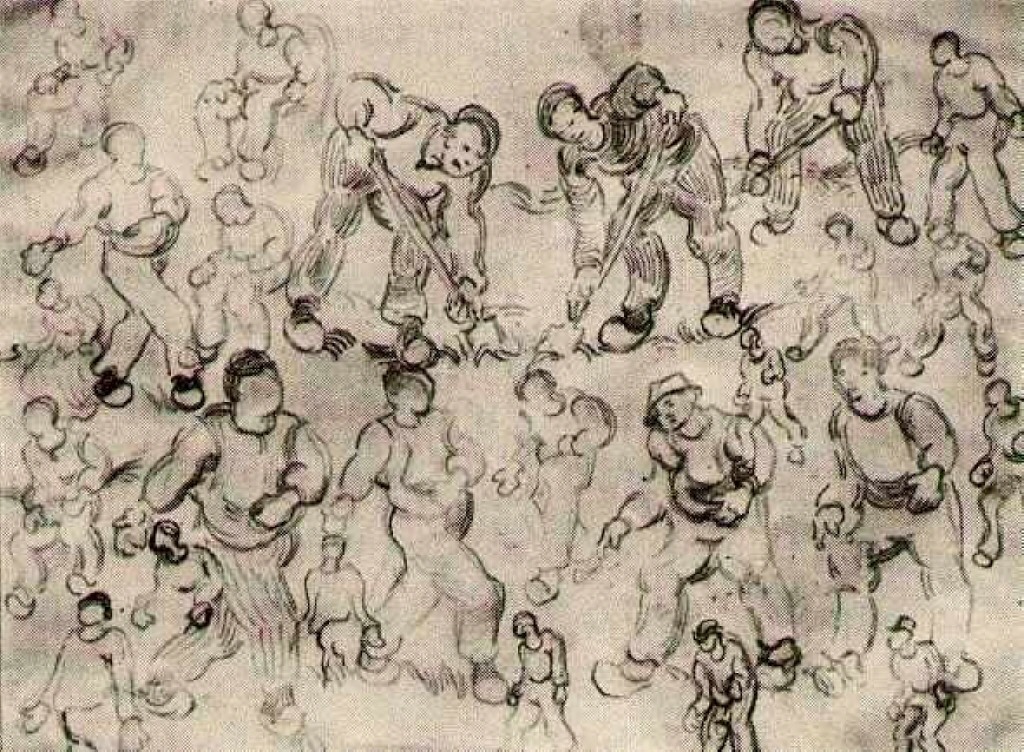This wide rectangular artwork appears to be a charcoal pencil drawing set against a beige-gray background. It intricately depicts various figures engaged in manual labor, their outlines rendered in a distinctly bubbly, exaggerated style. Prominently positioned at the top center are two nearly symmetrical men bent over, shoveling into the ground. To their left, faintly drawn individuals are seen sitting and throwing objects, while those on the bottom right are hunched over in various laborious tasks. At the bottom left, people march forward with unique, exaggerated strides. Although some figures are distinct with outdoor clothing and hats, many faces are left incomplete, merely circles, suggesting a study in movement and form. The scene is filled with figures of varying sizes, all characterized by their bulbous arms and shoulders, creating a dynamic and chaotic tableau of human activity.